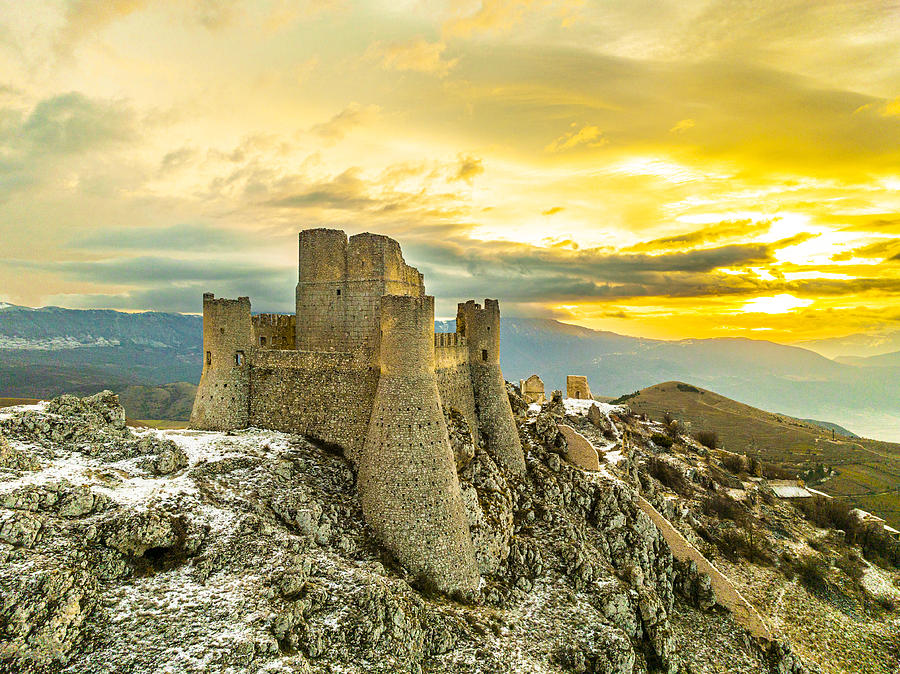The image captures a breathtaking sunset over a majestic mountaintop castle. At the top, the sky is adorned with a stunning blend of coral, white, and light gray clouds, with a bright, radiant yellow where the sun is setting. The clouds near the sun glow with an orange hue, adding warmth to the scene. Below this vibrant sky, the dark silhouettes of mountains or hills line the background. In the foreground, a grand, ancient castle stands proudly, its structure integrated into the rugged mountain terrain. The castle, built from brown, orange, and black stones, features turrets and square designs, suggesting it dates back several centuries. The rock formations supporting the castle vary in length due to the sloping mountain, with snow dusting the brown cliffs to the left. On the right, additional buildings and distant orange structures dot the landscape, adding depth to the mountainous vista.